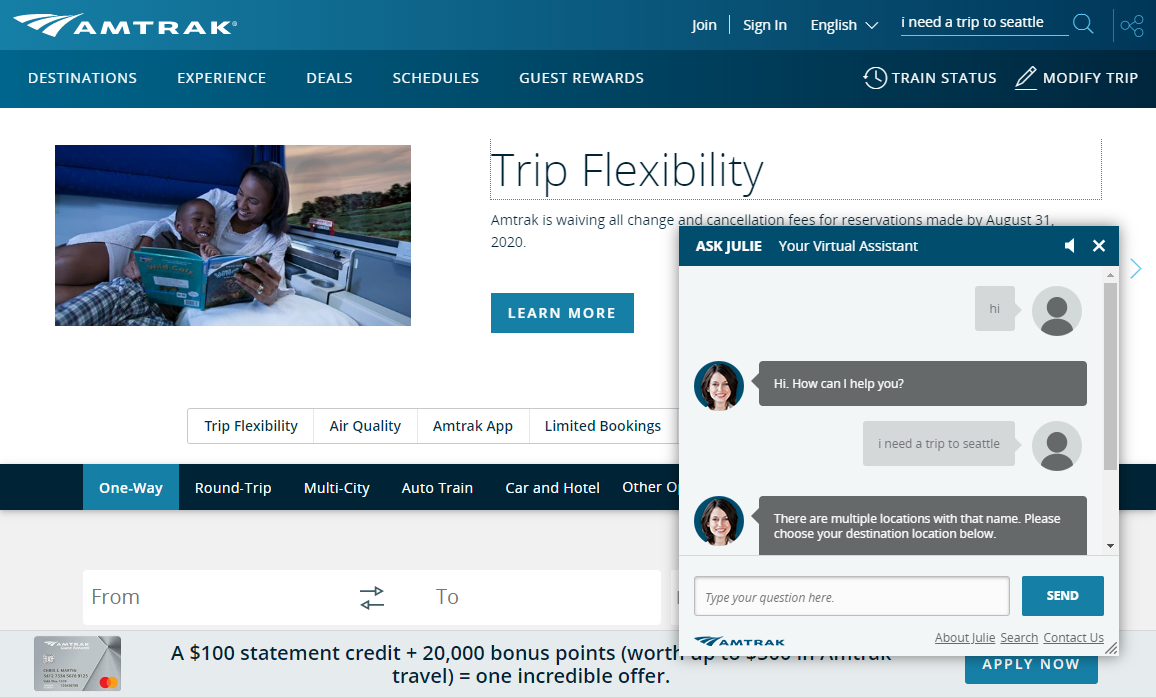The Amtrak website interface features a prominently displayed blue banner at the top, adorned with the Amtrak logo. The site offers options to join, sign in, and select your preferred language, which is currently set to English. Someone has already input a search query, "I need a trip to Seattle," indicating their destination. Below the search bar, navigation options including Destinations, Experience, Deals, Schedules, and Guest Rewards are available, along with sections for Train Status and Modify Trip.

A highlighted section titled "Trip Flexibility" is accompanied by a heartwarming image of a woman lying on a bed inside a train. She is reading a book to her pajama-clad child while the serene countryside rolls past the window. A caption informs users that Amtrak is waiving all change and cancellation fees for reservations made by August 31st, inviting them to learn more. Additional options listed under this section include Trip Flexibility, Air Quality, Amtrak App, and Limited Bookings.

In the travel booking area, the user has selected the "One Way" option, among others like Round Trip, Multi-City, Auto-Train, and Train and Hotel. They have engaged with Amtrak’s virtual assistant, Julie, by clicking on the chat bot. The assistant has asked how she can help and after the user's request for a trip to Seattle, the chat bot has responded noting there are multiple locations with that name, prompting the user to choose a specific destination before proceeding.

Overall, the user is navigating through the Amtrak website, actively engaging with its features, and seeking customer support for planning a trip to Seattle.